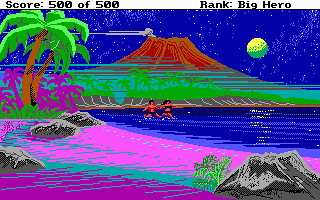A detailed in-game screenshot reminiscent of classic arcade aesthetics like Pac-Man, Gameboy, and Galaga, showcasing vibrant yet unconventional color schemes. The characters exhibit a unique reddish-orange skin tone, distinguishing them from traditional hues. At the top of the screen, the score is prominently displayed as "500/500" beside the rank titled "Big Hero," both in bold black letters with capitalized initials.

The scene captures a picturesque landscape featuring diverse elements: a verdant palm tree and grassland in the foreground, with a towering volcano under a star-studded night sky. The moon casts a gentle glow over the scenery, accentuating a small lake nestled nearby. Intriguingly, the beach is portrayed in a vivid purple, contrasting sharply with the blue sea. Central to the image are two characters, holding hands, their reddish-orange figures standing out against the colorful backdrop, creating an arcade scene brimming with nostalgic charm and imaginative detail.